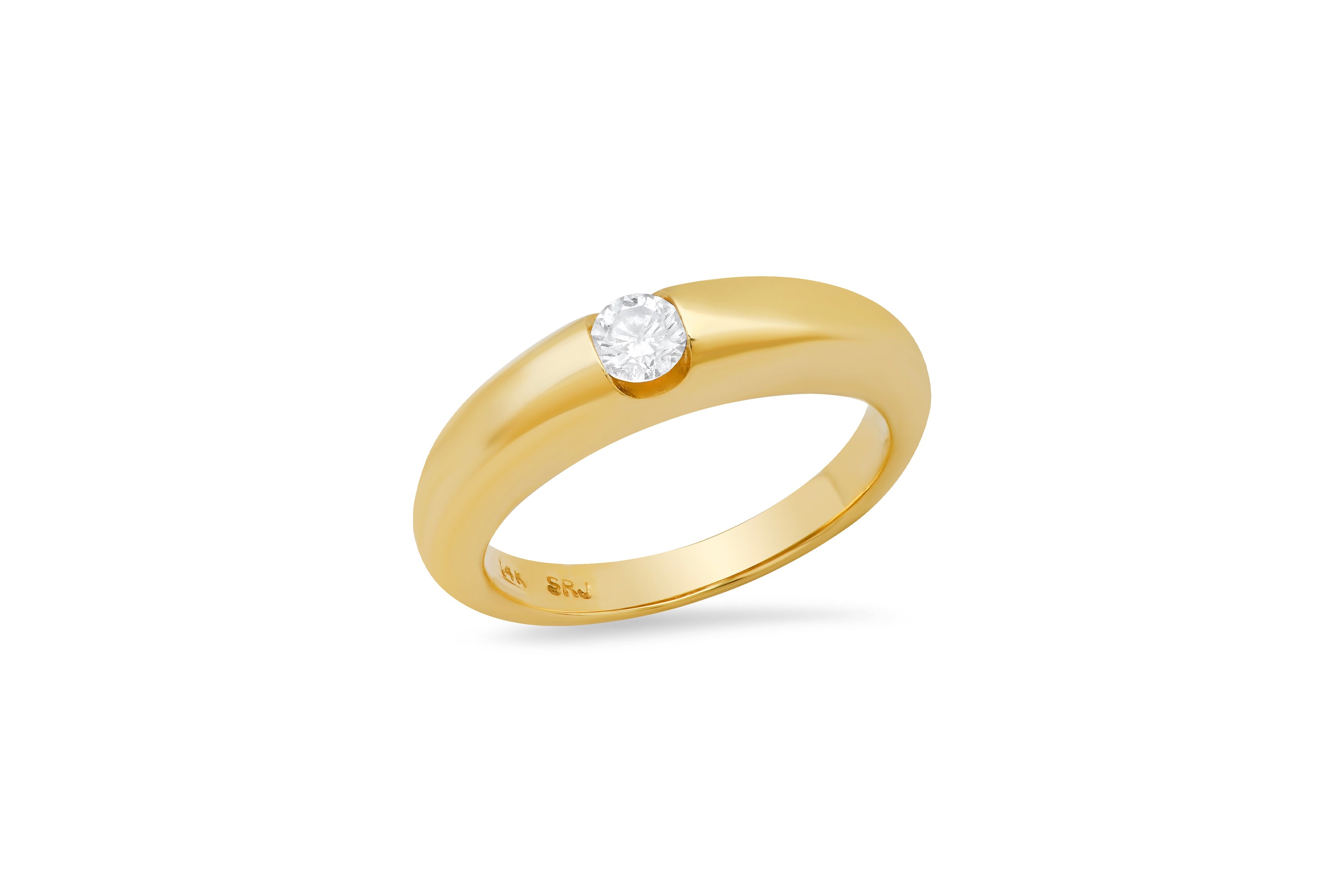This detailed product image showcases an intricately designed gold ring, potentially either a photograph or a highly realistic rendering. The ring features a single, prominent diamond embedded directly into its band, eschewing the traditional prong setting for a more integrated design. An engraving is visible on the inner surface of the ring, which appears to read "SRJ" with another indistinct word positioned above it. The ring is presented at an angle, allowing us to appreciate both the diamond set atop the ring and the inscription inside. The clean, white background ensures that the focus remains entirely on the ring's craftsmanship and unique features.